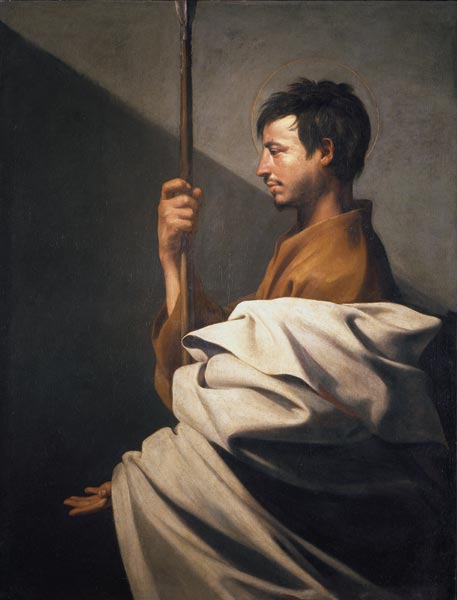This artwork, likely a painting or drawing, features a man positioned slightly off-center to the right within a vertical rectangular frame. The background is divided into two distinct areas: the upper portion features a medium gray triangle that stretches from the upper left to the middle right and back up to the upper right, while the lower segment transitions to a darker gray, almost charcoal.

The man, who has a medium complexion, is depicted in a contemplative pose facing left. He has short, slightly spiky dark brown to black hair, a thin mustache, and a small goatee. His eyes appear to be closed or nearly closed, suggesting a state of introspection.

His right arm is bent at the elbow and raised in front of him, holding a wooden pole or staff that extends out of the frame at the top. This pole is dark brown and suggests a spear-like object with a potentially metallic tip. His left hand is held below his waist, palm open, as if in a gesture of receiving or asking for something.

The man is dressed in a dark brown robe that covers his torso, with a white or light gray draped fabric enveloping his left side and arm, giving the appearance of a robe or cloak. This fabric casts shadows and folds, adding depth and texture to the image.

The background supports the composition, with the dark lower section contrasting against the lighter area above, enhancing the focus on the man who appears lost in thought.